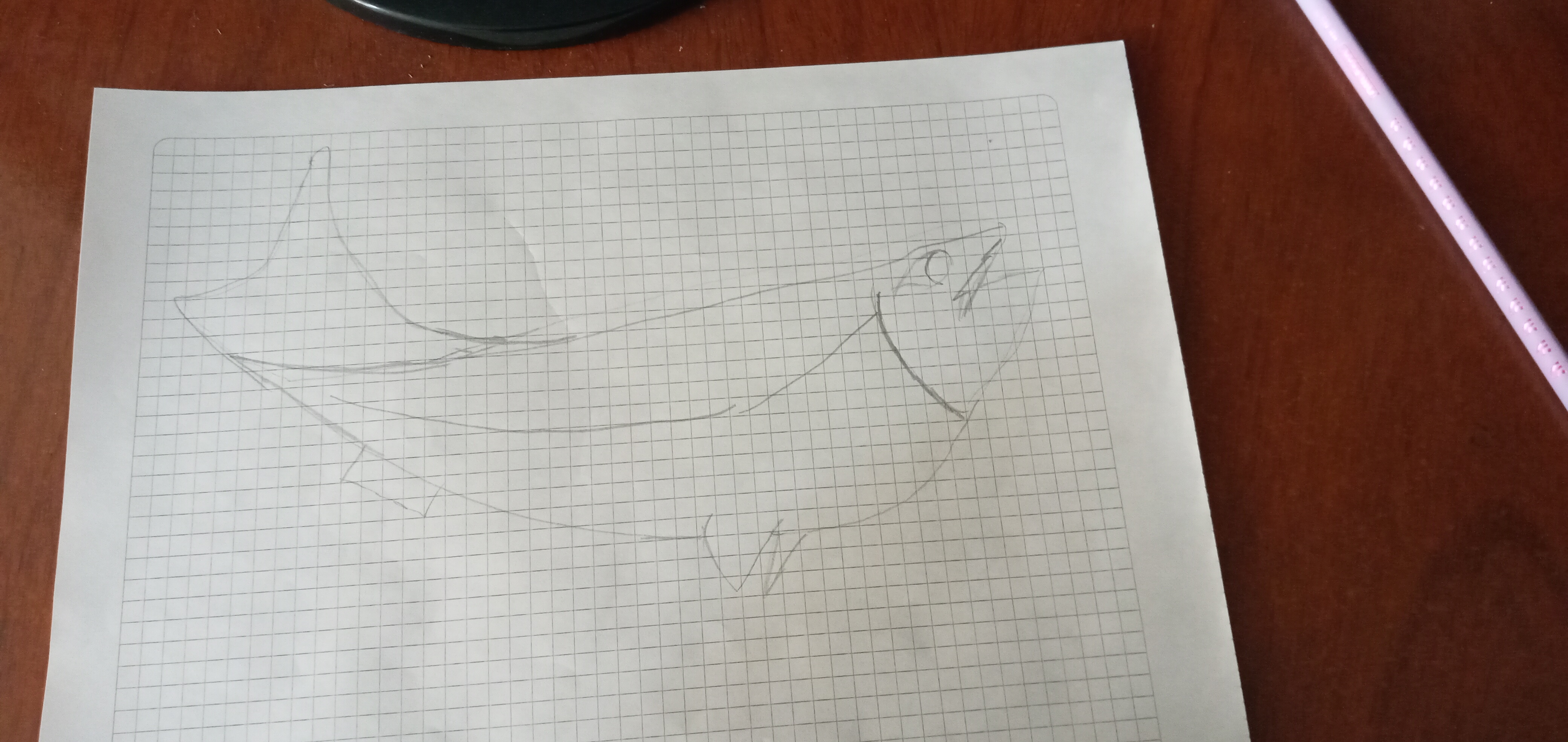A detailed caption for the image could be:

"A pencil drawing of a fish rests on a piece of white paper with a faint, small square grid pattern, resembling graph paper but with a noticeable white border around the edges. The artist utilized the grid to gauge proportions, resulting in a rough sketch where the fish is oriented to the right, its mouth open and body gently arcing downward and then upward to the left. The fish's tail is slightly notched, and the overall detailing is minimal. Situated on a brown wooden desk, the scene includes a pink writing instrument positioned in the top right corner and what appears to be a desk lamp or the black base of an object just above the paper."